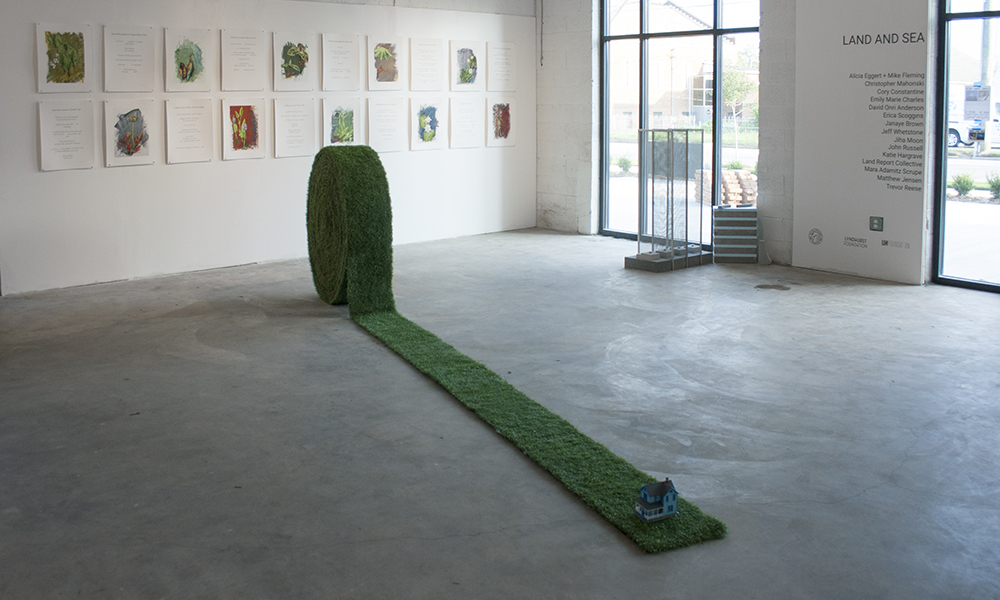This photograph captures the interior of a modern art exhibit space with pristine white walls and a polished concrete floor. The room features several black-framed windows through which a parked truck and greenery are visible, indicating a sunny day outside. Dominating the central wall are approximately ten paintings accompanied by ten sheets of paper with typed descriptions, potentially explaining the artworks. Along another wall, a prominent list titled "Landon C." showcases names including Alicia Eggert, Mike Fleming, Christopher Mahonsky, Corey Constantine, Emily Marie Charles, David Orie Anderson, Erica Scoggins, Janae Brown, Jeff “Whetstone” White, Gia Moon, John Russell, Katie Hargrave, and Land Report Collective.

A curious installation on the floor mimics a strip of green grass or turf, resembling a rolled-up hay bale or "fruit by the foot" with a coiled end. This green strip extends across the concrete and terminates in a small model blue house. The contrast between the artificial grass and the stark gallery environment highlights a playful yet thought-provoking aspect of the exhibit.